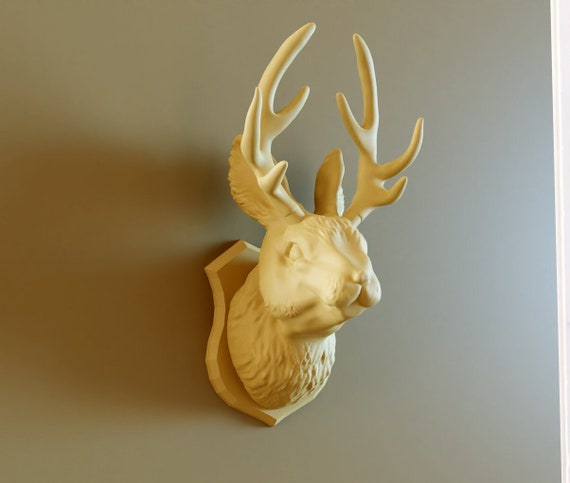This photograph features a meticulously crafted sculpture of a mythical jackalope, mounted on a shield-like wooden base. The piece artfully combines elements of a deer and a rabbit: it boasts large, branched antlers typical of a deer as well as the soft, endearing face and ears of a rabbit. The sculpture, rendered in an elegant, minimalist pure white or cream color, is intricately designed with lines accentuating both the head and the neck, giving it a refined, modern aesthetic. The jackalope is set against a plain, grey wall that enhances its sophisticated appearance, and it casts a distinct shadow to the left, adding depth and dimension to the display. This striking piece is a perfect example of contemporary art, blending whimsy and sophistication in a way that would be well-suited to a luxury home or a high-end art collection.